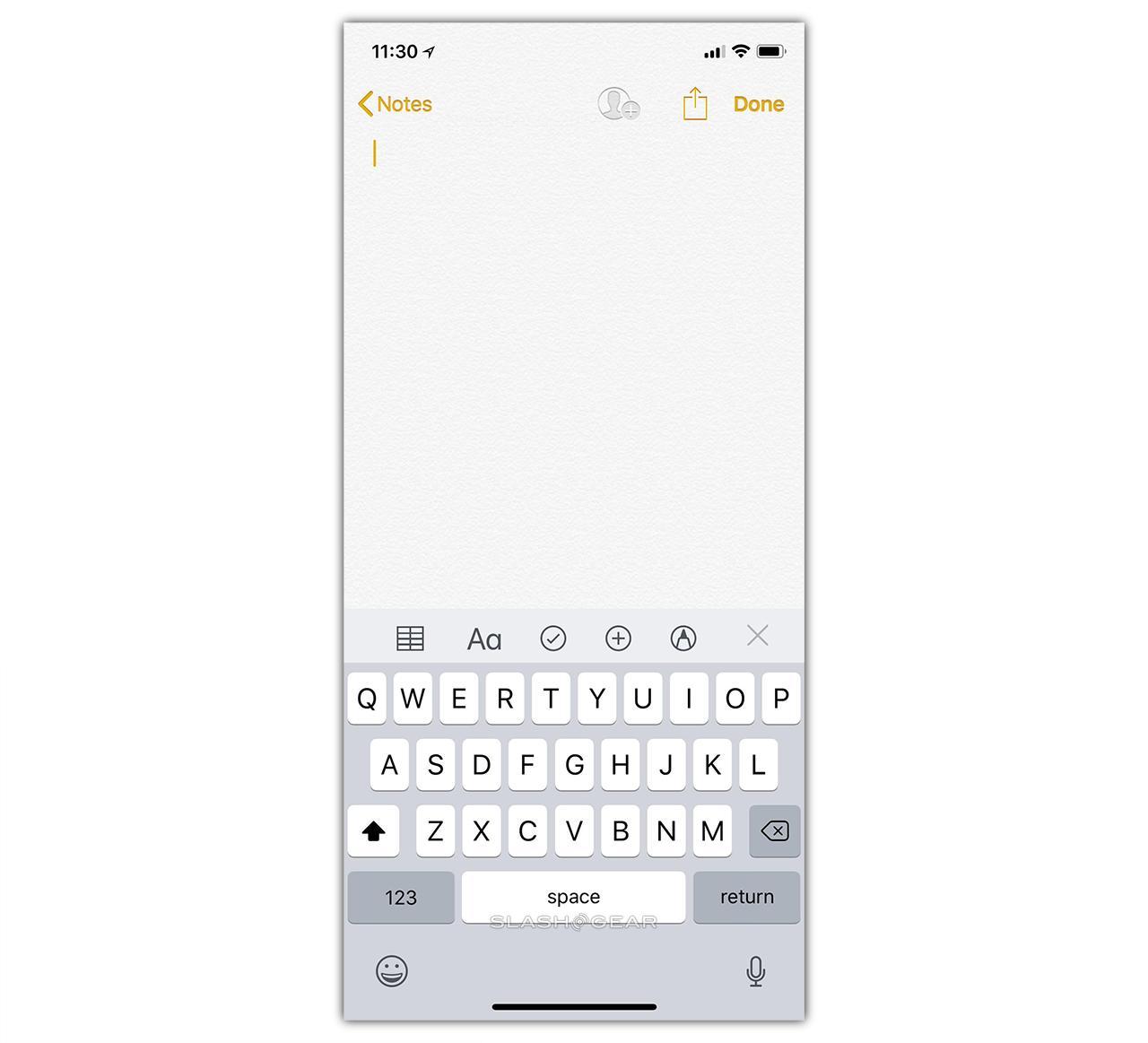Here is the cleaned-up and detailed caption for the image:

The image shows a cell phone screen displaying several interface elements. The top left corner of the screen indicates the time "11:30." On the top right, there are icons for cellular signal strength, Wi-Fi connectivity, and battery status, which reads as charged. 

Beneath these icons, there is a left-facing arrow next to the word "Notes" highlighted in an orangey-yellow color. Centrally located in the middle of the screen, there's a profile icon with a plus sign next to it, possibly signifying 'Add Contacts.' Beside this icon, there is a square with an upward arrow, commonly indicating a 'Send' or 'Share' function. The words "Done" and the square icon share the same orangey-yellow hue as the "Notes" label.

Below these options, there is a white text field with an orange cursor positioned at the top left corner. At the bottom of this field, there are multiple function icons: a table icon, a large 'A' and a small 'a' (possibly for text formatting), a circle with a check mark, a circle with a plus sign, a circle with a pencil tip, and an X mark.

Below the text field is a virtual keyboard. The keyboard keys feature white backgrounds with black text for the letters, while certain function keys like 'Backspace,' 'Return,' and '1 2 3' are gray. Centered over the spacebar is a watermark text that reads "/ clear gear /", which appears to have been added post-editing through a photo editor.

At the bottom of the virtual keyboard, a gray band is visible, housing a smiley face icon for emojis on the left, and a microphone icon on the right, likely for voice input.